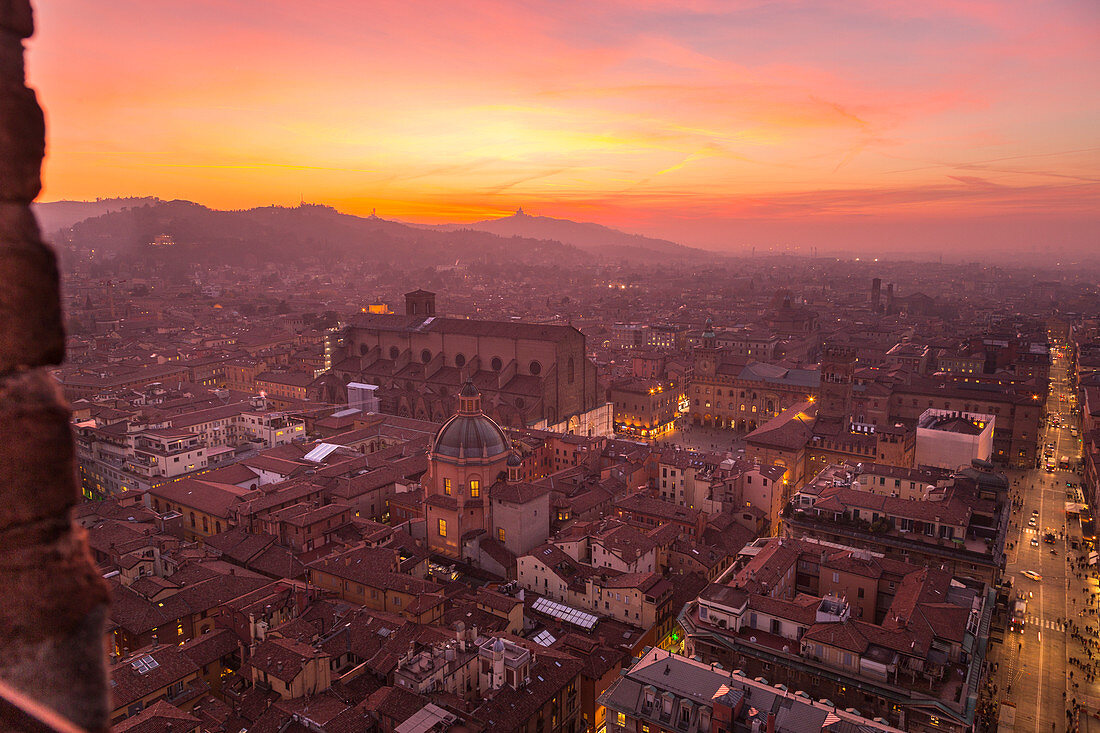The image presents a detailed, top-down view of a sprawling city, likely a rustic locale that could be in Italy or Spain, characterized by three to five-story buildings. The vantage point appears to be from atop a tall building, visible via a brick corner on the left side of the picture. Dominating the right side is a main street teeming with many cars, bordered by various side streets winding through the urban landscape. Toward the horizon on the left, a mountain range looms, with the sun setting behind it, casting vibrant hues of yellow, orange, and red across the sky, tinged with a hint of blue. In the foreground of the cityscape, a prominent building featuring a dome with a cross-topped spire stands out, suggesting it may be a house of worship. The scene captures a serene twilight setting, with indoor lights illuminating the architectural charm of this possibly religious town.